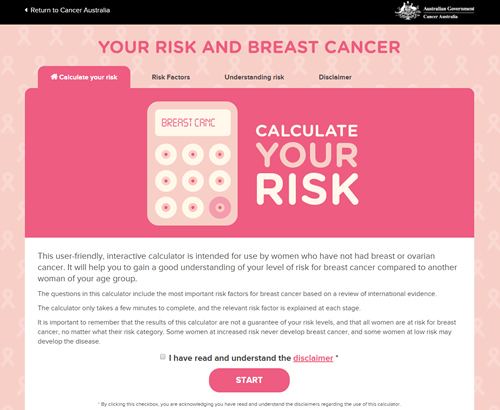The image depicts a website dedicated to assessing breast cancer risk, likely Australian as indicated by the mention of "Australia" and "return to cancer" in the text. The resolution of the image is notably poor, making some text difficult to read. Across the top of the website, there is a black strip featuring prominent white text that reads, “Your risk of breast cancer.” 

Beneath this headline is a navigation bar that includes options such as "Calculate your risk," "Risk factors," "Understanding risk," and "Disclaimer." The current tab selected is "Calculate your risk," highlighted in pink, while the other tabs remain in the standard background color with black font.

The main content area has a pink background featuring an interactive calculator in a lighter pink shade. The buttons on the calculator are white with a pink central area reminiscent of nipples. Adjacent to the calculator, “Calculate your risk” is prominently displayed. The calculator interface displays "breasts CAN" where numerical readouts would typically appear.

Below the calculator, the background is white and contains descriptive text. This text explains that the interactive calculator is designed to be user-friendly and is meant for women who have not had breast or ovarian cancer. It aims to provide a comparative analysis of an individual’s breast cancer risk relative to other women in the same age group. The description highlights that the included questions focus on key risk factors for breast cancer as identified through international research. The instructions clarify that using the calculator is a brief process.